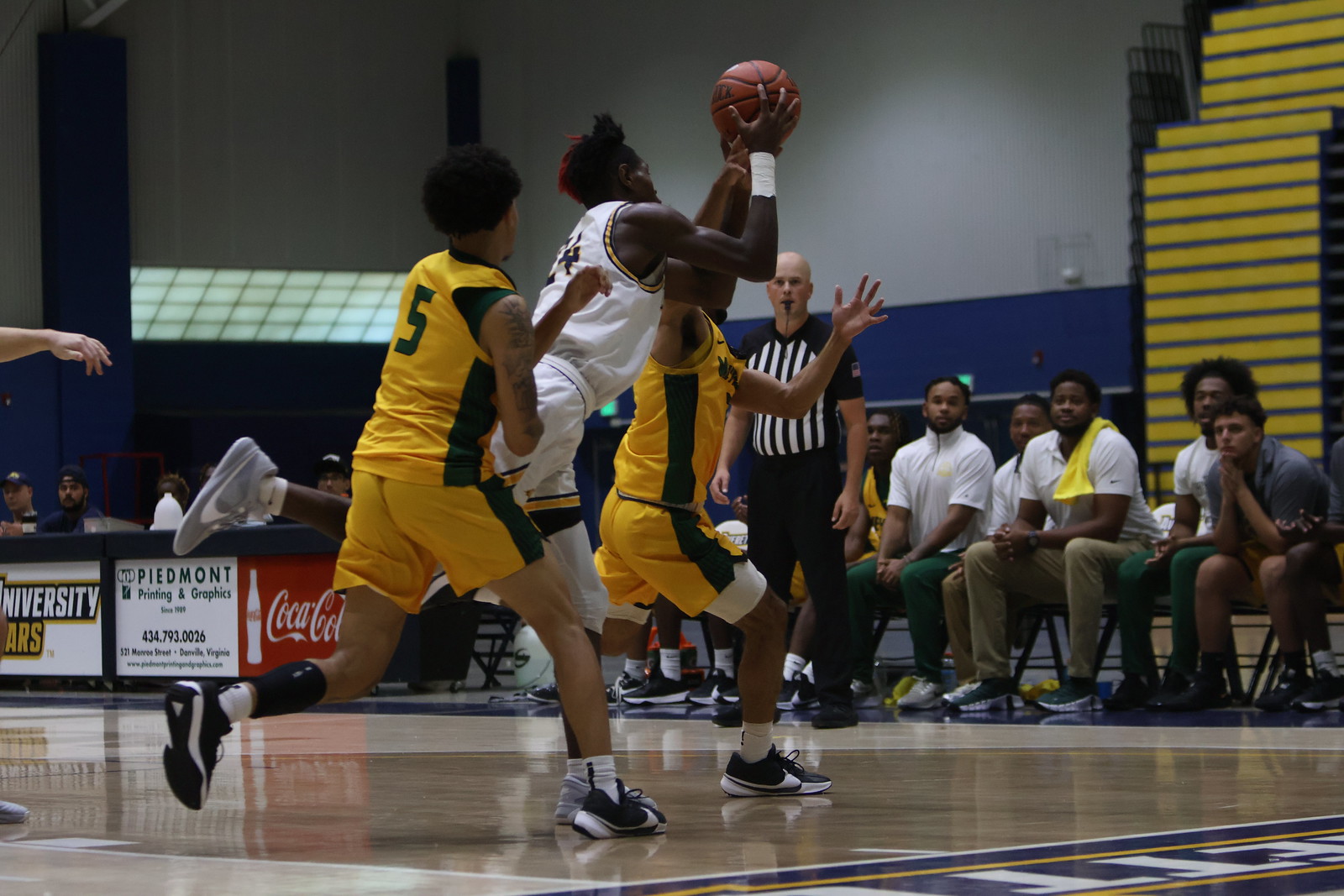In this high school gymnasium, the tense atmosphere of a basketball game is captured as players from opposing teams fiercely compete beneath the basket. Three players are in the spotlight: one in a white jersey and shorts attempts a shot, while two players in yellow jerseys and shorts with black stripes rigorously defend against him. The player in white is almost airborne, propelling himself forward with one foot off the ground, striving for a crucial basket. Meanwhile, one of the defenders in yellow, identified as number five, stretches his arms out in an effort to intercept the ball. Spectators fill the sidelines, watching the intense play unfold with anticipation. A prominent red Coca-Cola advertisement decorates the background, adding a splash of color to the scene, and the referee, dressed in black and white vertical stripes, closely monitors the action from the back.